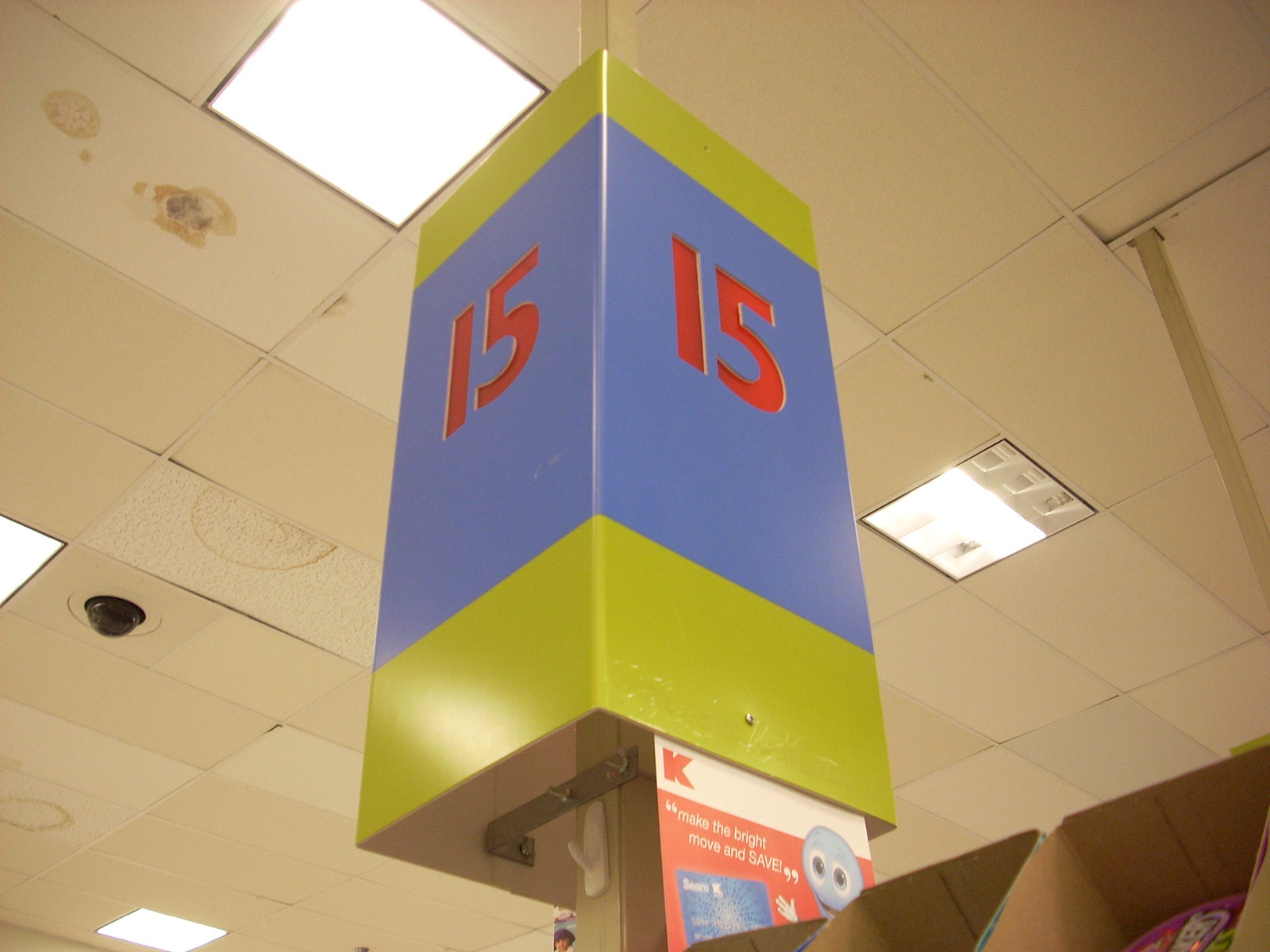The photograph depicts the interior ceiling of a grocery store aisle, specifically aisle 15. The ceiling is composed of beige, stained acoustic drop tiles, with embedded square white lights. A prominent green and blue aisle sign, with large red "15" digits and visible from all angles, hangs centrally from a pole. The ceiling also features various fixtures, possibly including smoke detectors or cameras, with one tile appearing blackened. In the lower right corner of the image, several cardboard boxes are visible, containing indiscernible items. Additionally, a Kmart promotional sign hangs from the ceiling, showcasing the store's red "K" logo, the slogan "Make the bright move and save," and a visual of a Sears and Kmart credit card, hinting at the store's past association with these brands. The overall scene feels dated and somewhat neglected.